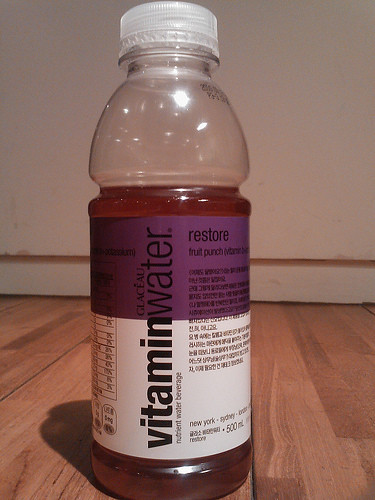This image features a plastic bottle of Vitamin Water, the brand name prominently displayed. The bottle has a smoothly rounded shape, with a clear cap and transparent body, showcasing a light reddish-brown liquid inside that fills about three-fourths of the container. The label is divided into two sections: the upper third is purple, while the lower two-thirds are white. The brand name "Vitamin Water" is written in bold, black lettering. At the top right of the label, the word "Restore" can be seen, followed by "Fruit Punch" and additional text that is not legible. The bottom part of the label indicates a volume of 520 milliliters. Part of the nutrition label is visible on the left side of the bottle. The bottle is placed on a light brown wooden floor, with a white wall in the background.